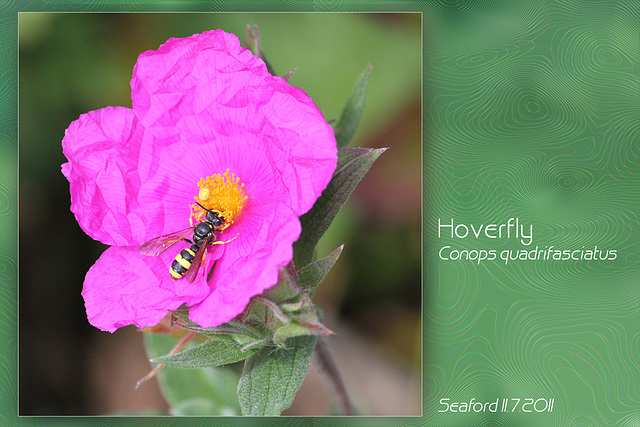The image features a vibrant and vivid pink flower with crumpled petals and a yellow center, displaying golden pollen. Beneath this pollen, a large bee with a black body and distinctive yellow-and-black striped tail can be seen, its wings visible. The flower is accompanied by green leaves, adding depth to the scene. The background is a bright, blurred gradient of green with subtle wavy coils. On the right side of the image, text in white indicates "Hoverfly Conops quadrifasciatus," and below this, "Seaford 27-2011." This composition suggests a moment of natural pollination, captured in a nature-themed photograph.